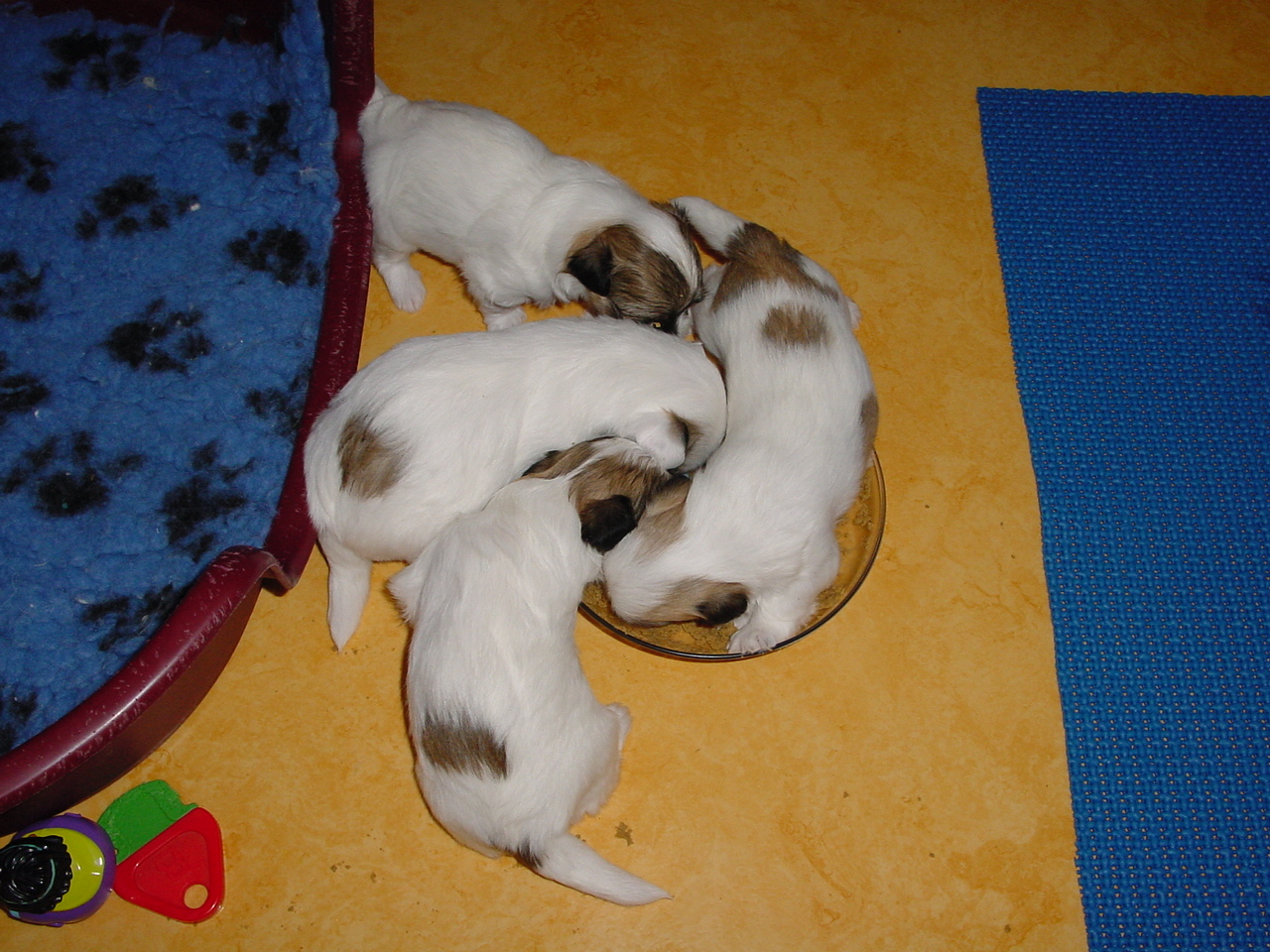The image captures a scene of four recently born puppies, predominantly white with brown spots and brown ears, nestled together in a big glass pie plate on a yellowish floor with a swirl design. The puppies are curled up in a semi-circle, their tiny faces touching, and one of them is standing in the bowl, pushing in to join the others. To the left of the image, there is a maroon-colored dog bed with a blue blanket patterned with black paw prints, and nearby are two chew toys—a red and green mushroom toy and a yellow ball with purple accents. To the right, partially off-frame, lies a blue mat. The puppies, still small and adorable, look cozy and peaceful in their snug arrangement.